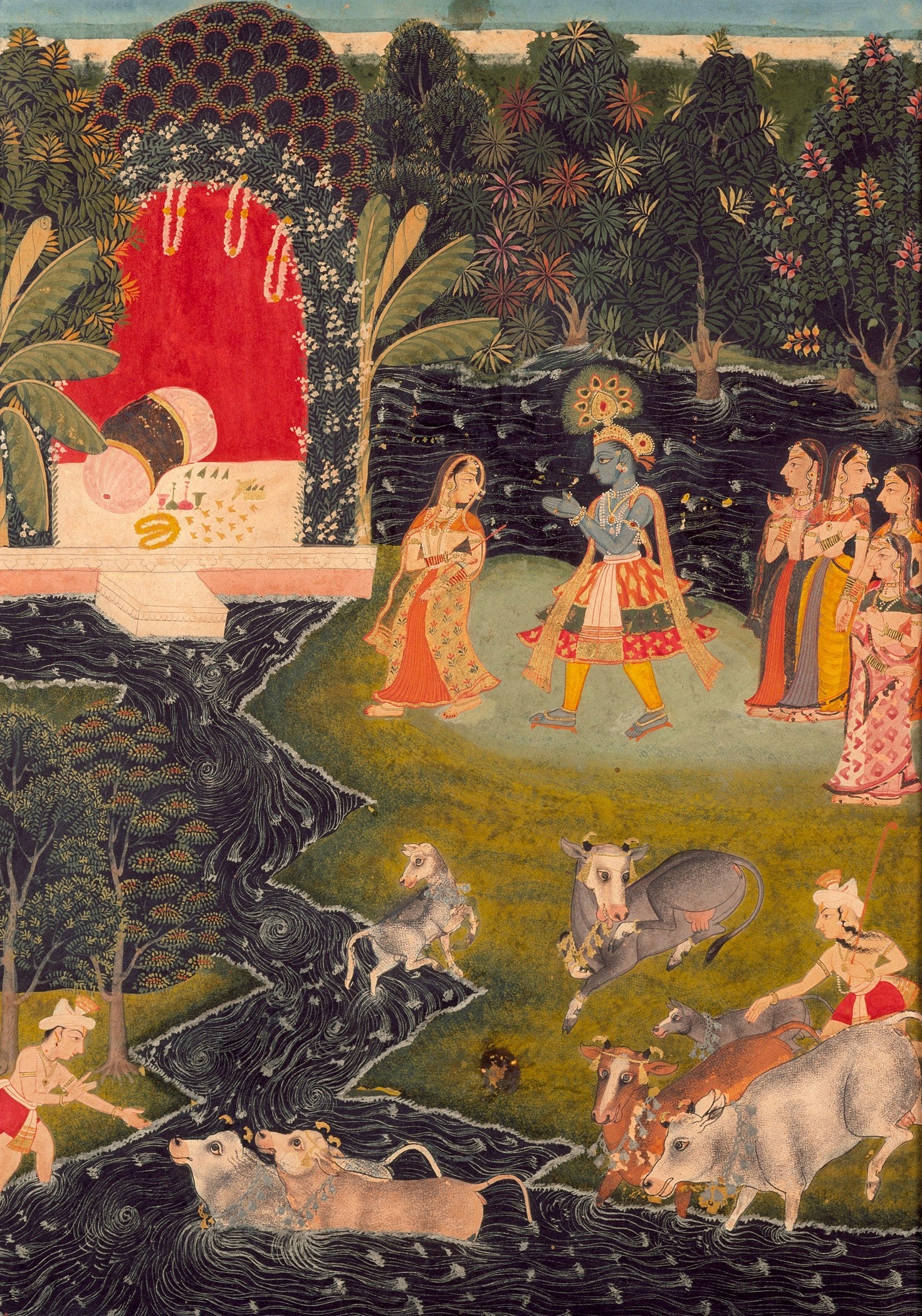This Indian or South Asian style painting presents a vibrant and detailed scene set against an outdoor backdrop. At the center is a striking figure of a blue-skinned man, adorned in elaborate attire, including numerous white necklaces, a tutu-style layered dress, yellow pants, and sandals that reveal his blue feet. His headdress is decorated with bejeweled peacock-like elements. His hands are gesturing forward, suggesting movement or instruction. Surrounding him are several women, characterized by their long pointy noses, wide flat eyes, and long dresses with multi-colored patterns. Some wear hair coverings.

In the foreground, a small structure can be seen in the top left corner, featuring a bed with a large pink pillow and an archway entrance, framed by a picturesque setting of plants and trees. Below this structure flows a river, painted with blue and white swirls in a zigzag pattern, indicating water's movement. 

In the lower section of the painting, a man in a red loincloth and pointy white hat tends to two cows in the river, with another similarly dressed man and additional cows, along with a gray dog, in close proximity. The river, lush greenery, and livestock contribute to the serene, yet bustling narrative of the artwork, which balances artistic representation and recognizability without striving for naturalism.